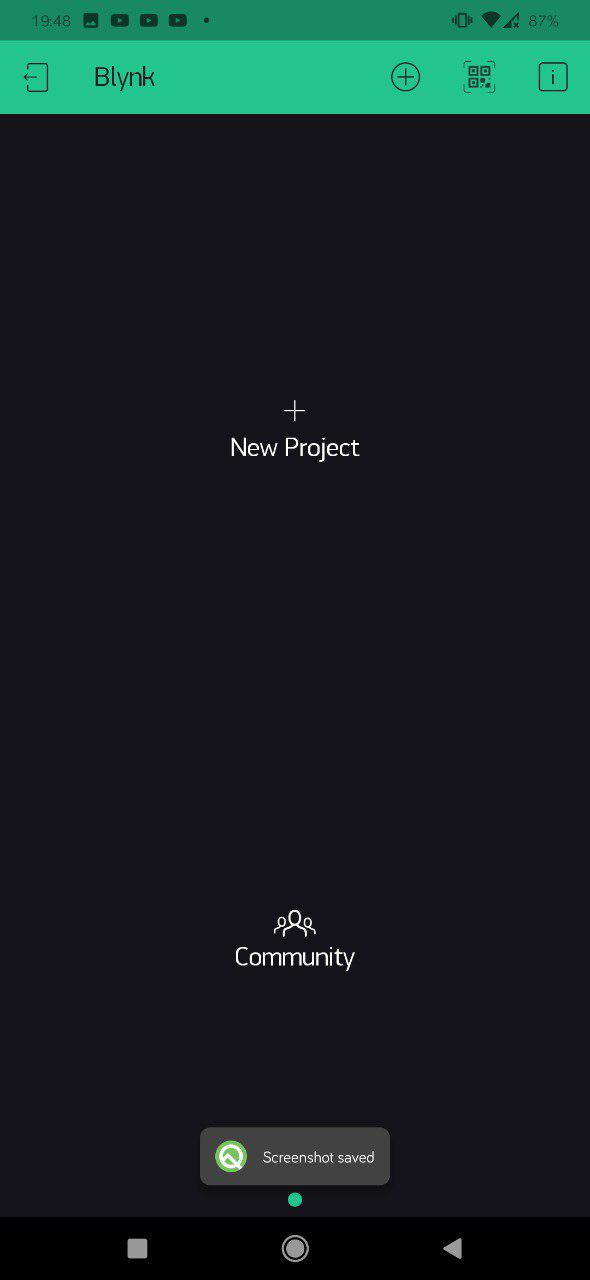The image is a detailed screenshot of the mobile app "Blynk," spelled B-L-Y-N-K. The top header has a green color background, prominently displaying the app's name, "B-L-Y-N-K." Alongside, on the far right of the header, there are three icons: a plus sign (+), a square with an 'i' inside of it, and another unspecified icon. 

The body of the app's interface is predominantly black, featuring a centrally placed plus sign (+) accompanied by the text "New Project." Towards the bottom center of the screen is a community section represented by the text "community" and an icon depicting the outline of three individuals. 

The footer of the screenshot includes a notification box displaying "Screenshot Saved." The time on the mobile device is indicated as 19:48, shown at the top left corner. On the top right corner, the battery level is 87%, alongside several other status icons including the cellular signal, data connectivity, and a vibrate mode indicator.